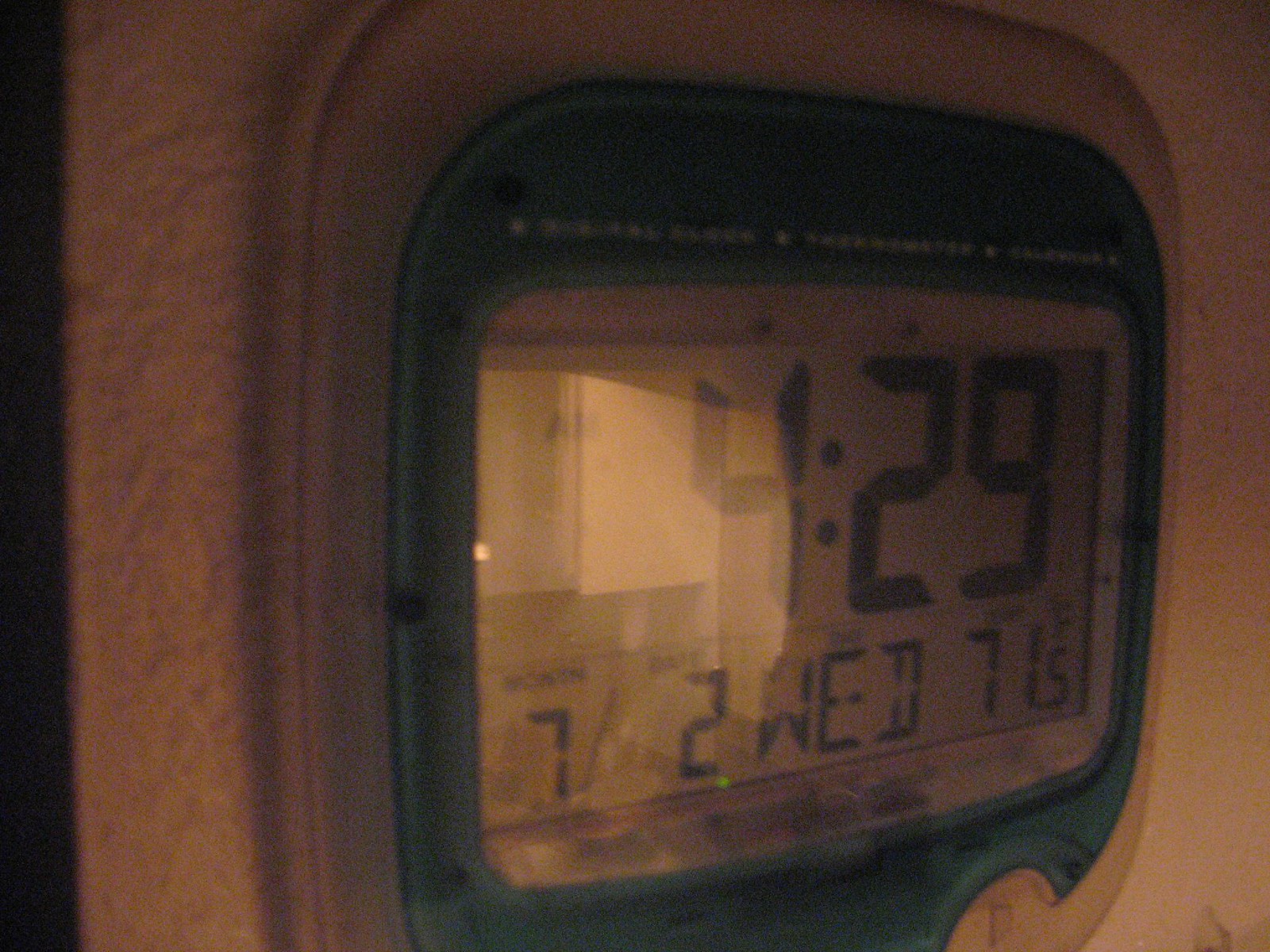In this close-up image, a small, square-shaped digital clock is prominently displayed, mounted on a white wall. The clock features a thick, silver outer frame encasing a slightly smaller green-bordered square. The central digital screen has a gray background with black digital numerals displaying the time as 4:29. Below the time, smaller digital readouts indicate additional information: the month ("7"), the date ("2"), the day ("WED"), and the temperature ("71.5°F"). The clock is captured from a side angle, resulting in a partial light glare across the digital screen, likely caused by a nearby lamp. This gentle illumination adds a subtle sheen to the display, enhancing the clock’s metallic and digital elements.